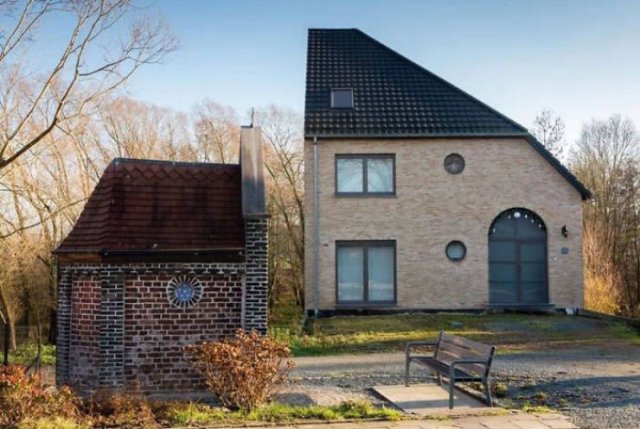The image depicts two buildings against a clear blue sky with bare-branched trees suggesting it's fall or winter. On the right half of the image, there's a two-story house that looks as if it were sliced down the middle. It has a beige exterior composed of light and medium brown bricks or stones. The house features two rectangular windows and two smaller circular windows. An arched, dark gray front door sits on the right side, beneath a black tiled roof with an air vent protruding from it. The house also includes a small window at the top of the roof.

On the left side of the image, positioned in the foreground, is a smaller building reminiscent of an outhouse. This structure is built of reddish-brown and white bricks and has a small, dark brown sloped roof with a chimney. A circular decoration is visible on its front. 

In front of and to the right of the smaller building is a wooden bench on a concrete slab, facing the small building. The bench sits amidst a gravel driveway and patches of grass, some of which contain dead bushes. The scene is outdoors, likely a residential area with hints of greenery and sparse foliage, characteristic of late autumn or winter.